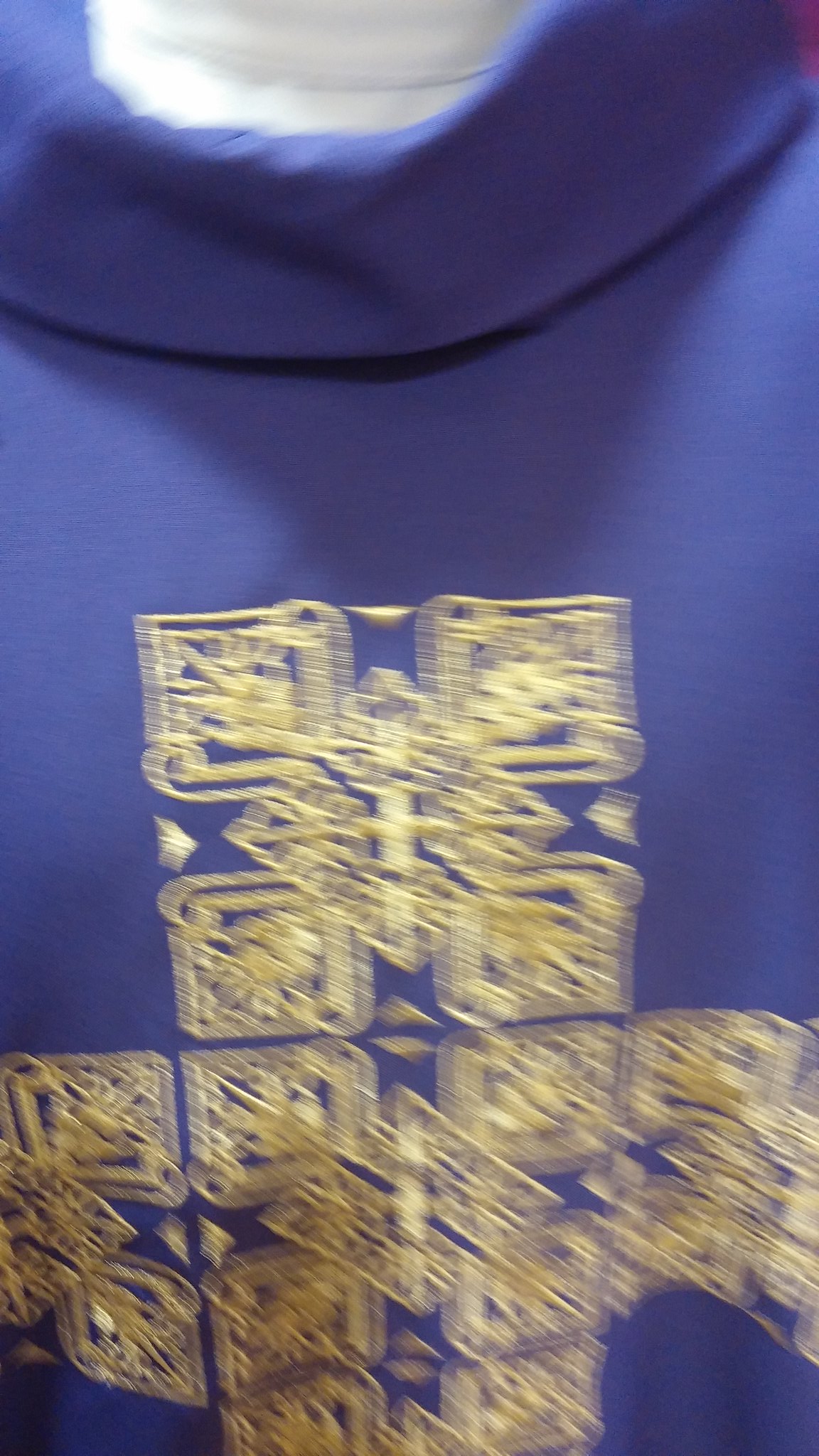This image depicts a blurry, out-of-focus photograph of a purple sweatshirt, likely displayed on a mannequin with a white plastic neck. The sweatshirt features an elaborate gold filigree design forming a cross on the front, comprised of repeating square patterns with diamond shapes in between. The background showcases blue and purple hues, adding contrast to the intricate golden ornamentation. The garment appears to have a unique, loose turtleneck style, differing from a typical hoodie. Though the details are somewhat hard to discern, the sweatshirt's distinctive open-neck design and ornate golden cross pattern are prominent.